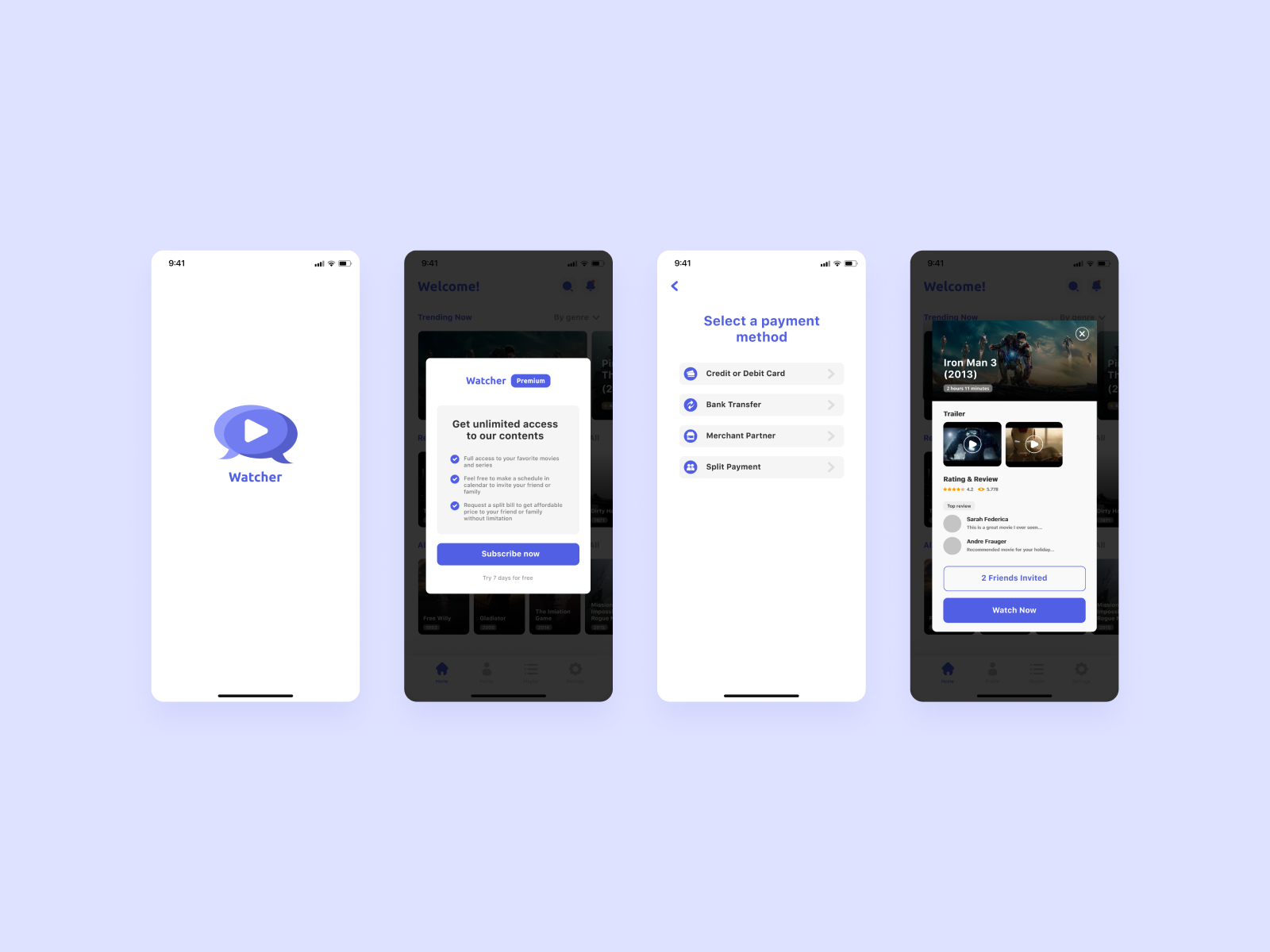This rectangular color image features a horizontal layout with a bluish-light gray background. It showcases four distinct cell phone screen captures, each highlighting different app interfaces. 

On the far left, the screen display has a white background, prominently featuring a chat bubble with a solid white arrowhead pointing to the right. Inside the chat bubble, the word "Watcher" is displayed in light blue-purple letters. 

The next screen to the right presents a black background with a prominent white rectangle at its center. The word "Watcher" appears again in light purple text. Below it, a light purple-blue filled bubble with the word "Premium" is visible, along with the text "Get unlimited access to our contents." Further down, three blue dots contain white check marks.

The third screen captures a payment method selection page, listing four different options: Credit or Debit Card, Bank Transfer, Merchant Partner, or Split Payment.

Finally, the screen on the far right is an advertisement for the movie "Ironman 3" (2013), which offers two call-to-action buttons at the bottom: "Watch Now" or "Invite Two Friends."